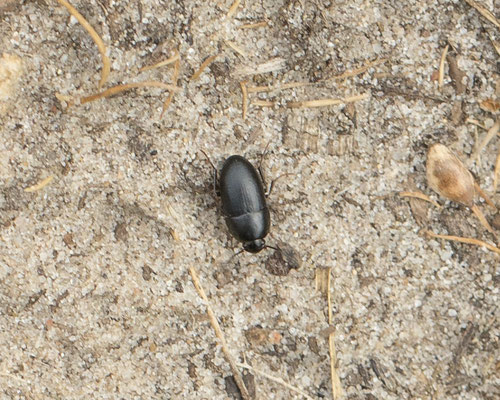The image features a detailed close-up of a black beetle with a hard, oblong shell, distinguished by a small line where its shell articulates. The beetle's head is adorned with two antennae. It crawls across a sandy, beige-colored ground that features diverse shades of brown, ranging from medium brown to whitish-brown. The sand is mixed with smaller rocks in similar tones and is scattered with dead grass, resembling fine straw, along with some dead leaves or stems. Additionally, the image is horizontally rectangular, and in the top right corner, there is a larger brown object that may be the shell of a dead beetle. The beetle appears to be moving forward, creating a dynamic sense of motion amidst the trampled-down field-like background.